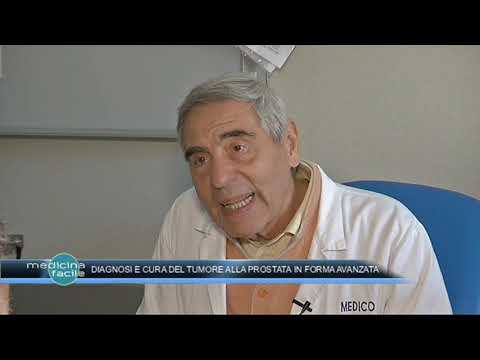The image features an older gentleman, possibly in his late 60s, with gray hair and a touch of black, seated in a blue office chair. He appears to be speaking, with his mouth slightly open, and is wearing a white doctor coat over a coral-colored button-down shirt. The name "M-E-D-I-C-O" is printed on the left side of his coat. A microphone is clipped to his jacket, suggesting he is being recorded, likely for a television show or news program.

The background is neutral, with a whiteboard and a tan or white wall behind him. The picture is flanked by horizontal black bars at the top and bottom. There is a text bar at the bottom of the image, consisting of a solid dark blue band with lighter blue bands above and below it, and a teal circle at the start. The white text within this bar reads "Medicina Facile" and "Diagnosi e cura del tumore alla prostata in forma avanzata," which translates to "Diagnosis and Treatment of Prostate Cancer in Advanced Form" in English.